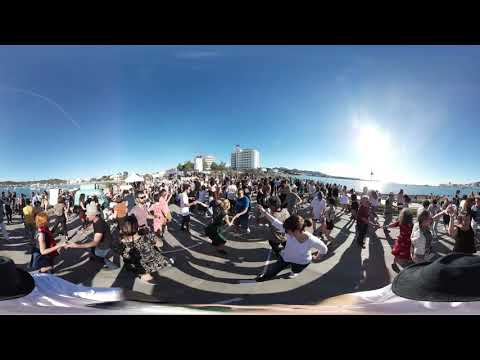This image captures an outdoor scene, likely taken with a wide-angle lens or in panoramic mode, which has contributed to a warped and somewhat distorted appearance. The setting includes a large crowd of people, possibly numbering in the hundreds, gathered on a gray, paved patio structure. They are engaging in various activities such as dancing, mingling, and walking around. The bright sunlight casts elongated, curved shadows on the concrete due to the angle at which the photo was taken. 

In the background, a serene stretch of water—either a lake or a river—reflects the low sun, which is positioned to the right and illuminates the entire scene. The sky is a stunning blue, transitioning to a lighter hue near the horizon. A tall, white high-rise building, possibly an apartment complex or hotel, stands prominently among a cluster of smaller buildings. Green trees are visible, adding a touch of natural beauty to the landscape. The scene appears to be taking place on what might be an island or coastal area, enriched by the clear weather, making it a picturesque day. People are dressed in light, casual clothing appropriate for a sunny day, enhancing the overall vibrant atmosphere.